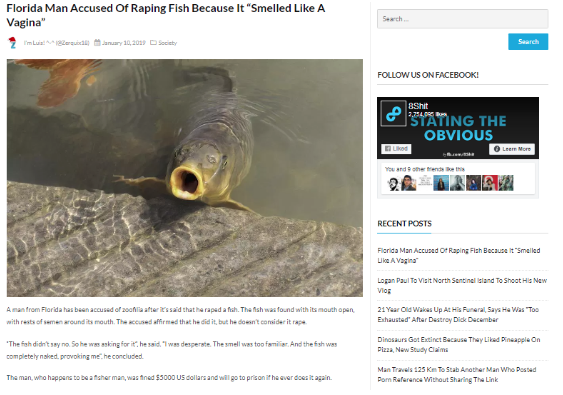This image from a computer screen captures a snippet of a bizarre and distressing news article. The main headline reads, "Florida man accused of raping fish because it smelled like a vagina," and features an accompanying image of a fish. According to the article, a Florida resident, described as a fisherman, has been accused of zoophilia after admitting to sexually assaulting a fish. A photo shows the fish with its mouth open and a visible presence of semen around its mouth. The man reportedly claimed that he did not consider his actions to be rape, stating that the fish did not say no and implying that it was 'asking for it' due to its smell and lack of clothing.

The man justified his actions by saying he was desperate and provoked by the fish, adding that the familiar scent had driven him to commit the act. For his actions, the fisherman was fined $5,000 and warned that he would face imprisonment if he repeated the offense.

To the right of the article, there are various online elements, including a section titled "Stating the Obvious," a prompt to follow the publication on Facebook, and a search area. Below these, there is a clickable link to another article about Logan Paul planning to visit North Sentinel Island for a new vlog. Additional articles are listed underneath, including one titled "21-year-old wakes up at his funeral, says he was too exhausted after 'Destroy Dick December.'"

The screenshot provides a snapshot of a sensational and disturbing piece of news, alongside other unusual story headlines.